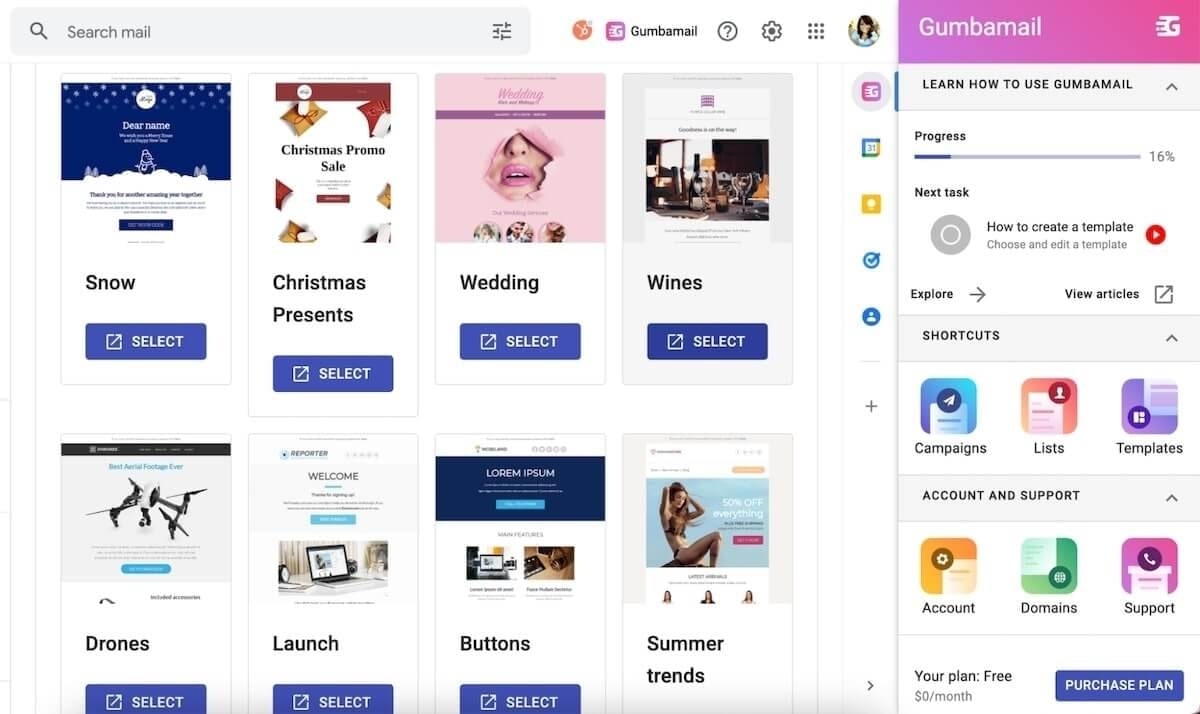Here's a detailed and cleaned-up caption for the image:

---

This image is a screenshot of the Goomba Mail app. On the far right is a sidebar with a pink header that displays "Goomba Mail" in white text and a "G" logo in the upper right corner. This section includes a progress bar currently at 16%. Below the header, there are sections for shortcuts and account management. The shortcuts section features three icons labeled "Campaigns," "Lists," and "Templates." The account and support section includes icons for "Account," "Domains," and "Support." At the bottom of the sidebar, there's a note indicating the current plan: 'Your plan: Free - $0/month,' along with a blue "Purchase Plan" button.

Dominating the left side of the webpage, which serves as the main body of the app, is a functional area with a white background. The top left corner houses a mail search bar. Adjacent to this, extending towards the right, are icons for Goomba Mail, help (question mark), settings (gear), and a user profile, which appears to represent a female user.

The main content area showcases eight distinct templates, each within its own box and each featuring a blue "Select" button at the bottom. 

- **Snow**: The first template on the left has a theme of white ground beneath a blue sky with falling snow.
- **Christmas Presents**: The second template has a white background with a "Christmas Promo Sale" banner in the middle and a red button below it. The template also includes images of Christmas gifts adorned with red bows and has a red header.
- **Summer Trends**: The last template in the second row shows a model in a tank top and boy shorts, seated on a beach, embodying a summer theme.

---